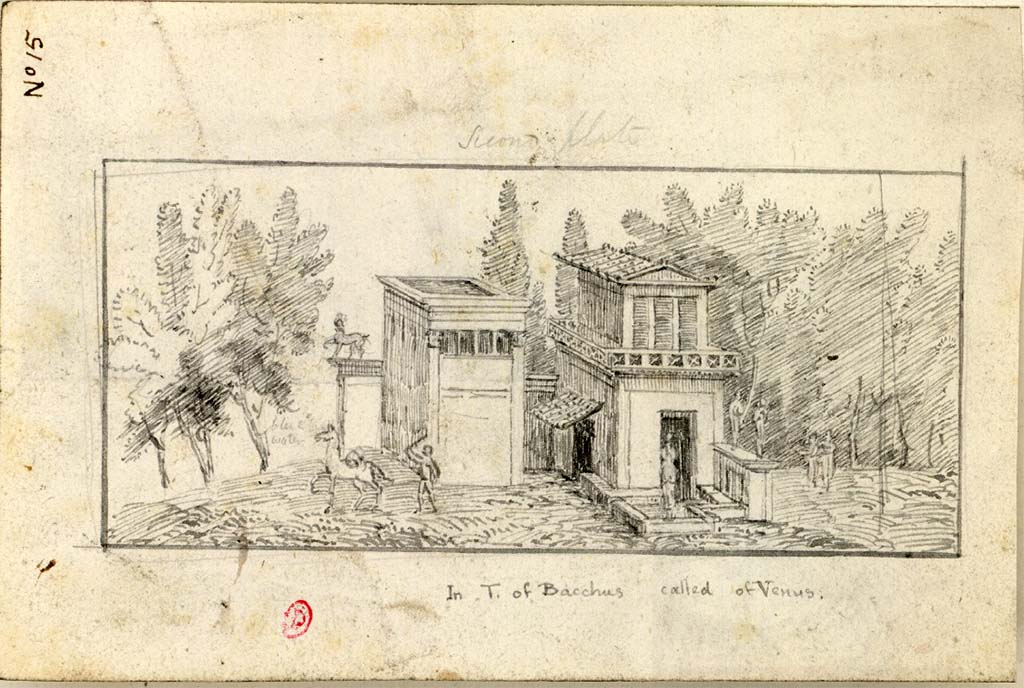A very old and weathered sketch, printed on what appears to be aged white paper, now almost brown due to its antiquity. The piece is horizontally rectangular with faint brownish smudges which might be dirt or simply part of a secondary paper beneath it. In the upper-left corner, the handwritten text states "No 15" in black, oriented sideways. Unidentifiable cursive writing, possibly in gray pencil, is scribbled above and below the main image. A distinctive red mark, specifically a "D" with a circle around it, is noticeable at the bottom left. Beneath the drawing, the inscription reads "T of Bacchus, called of Venus."

The centerpiece features a black rectangular border enclosing a black-and-white scene. In this scene, two buildings are depicted: the left possibly a storage place or garage, and the right a two-story house with large front entrance and windows extending to the back. A man is visible whipping a horse in front of one building. There's another animal, possibly a dog, on the deck. Gray and white trees sketch the background on both sides, and additional people are scattered across the scene, all rendered in the same graphite texture. The overall sky and ground are filled in with gray sketching, unifying the composition in this delicate and meticulously detailed historical artwork.